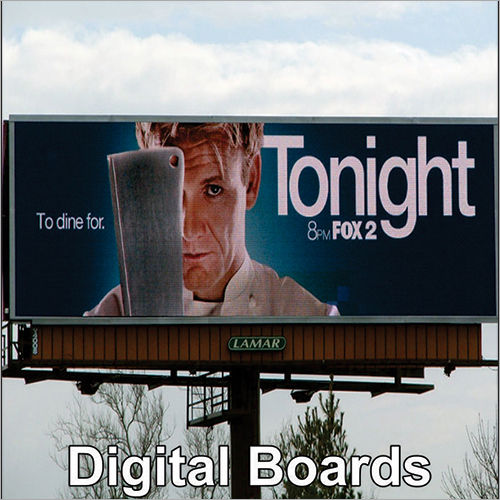The image showcases a digital billboard managed by Lamar, set against a backdrop of trees and a partly cloudy sky. Prominently featured on the billboard is Chef Gordon Ramsay, depicted holding a cleaver that obscures part of his face, giving a serious look towards the viewer. To the left of his image, in white text on a royal blue background, the slogan reads "To Dine For." To the right, larger text announces, "Tonight, 8 p.m., Fox 2," indicating the broadcast time for one of his television shows. The lower portion of the photograph includes an overlay of the words "digital boards," emphasizing the dynamic nature of the billboard. The color palette of the image includes sky blue, white, royal blue, beige, green, and yellow.